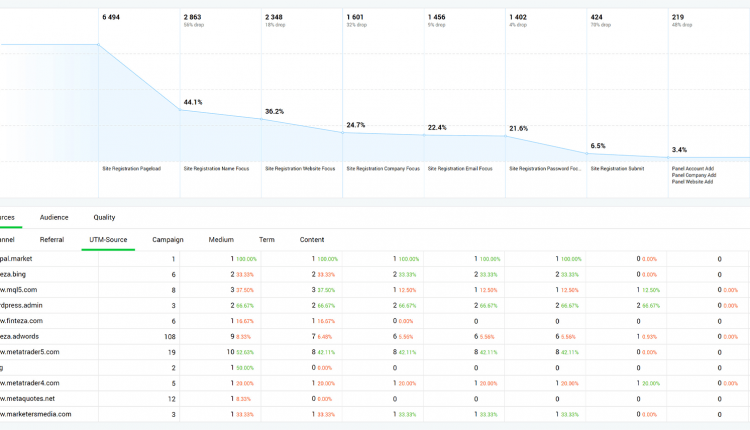The image showcases a detailed computer-generated graph and table. At the top, a blue line graph is prominently displayed, illustrating a progressive decline from a high starting point, steadily decreasing to a significantly lower value by the final mark. The graph is annotated with numerous percentages and numerical values, indicating various categories.

Beneath the graph, there is a comprehensive table divided into rows and columns, resembling a spreadsheet. This table includes columns labeled "Audience," "Quality," "Referral," "UTM," "Campaign," "Medium," "Term," "Content," "PAI Market," "ECZ," and "Bing," presumably representing different datasets or stock names. The table entries comprise a range of numbers, including frequent ones and twos, occasional sevens and eights, and values reaching up to 108 in certain sections. The overall layout provides a thorough analytical overview, combining visual and numerical data for detailed examination.